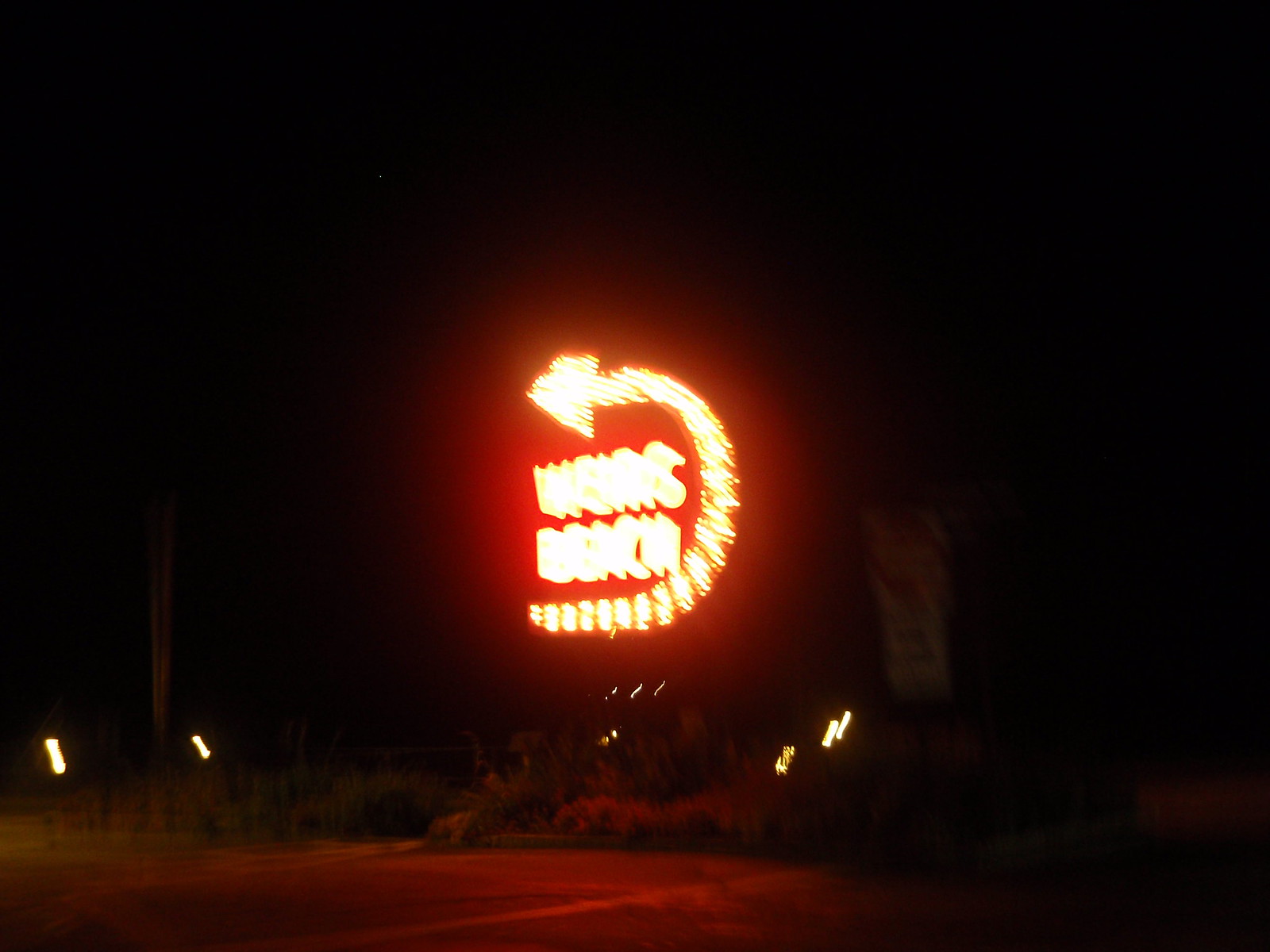In the image, a dimly lit scene makes it difficult to discern the surroundings. However, at the very center, a brightly illuminated sign commands attention despite being partially obscured by its intense glow and a slight blur in the image. The lights on the sign emit a striking red-orange hue. The sign features two words, though the brightness makes the top word unreadable. The lower word clearly reads "BEACH." Below "BEACH," the tail end of an arrow curves up and over the obscured top word, ultimately pointing to the left side of the image. In the foreground, faintly illuminated pavement or a parking lot is visible. The background fades into complete darkness, adding to the overall mysterious ambiance of the scene.